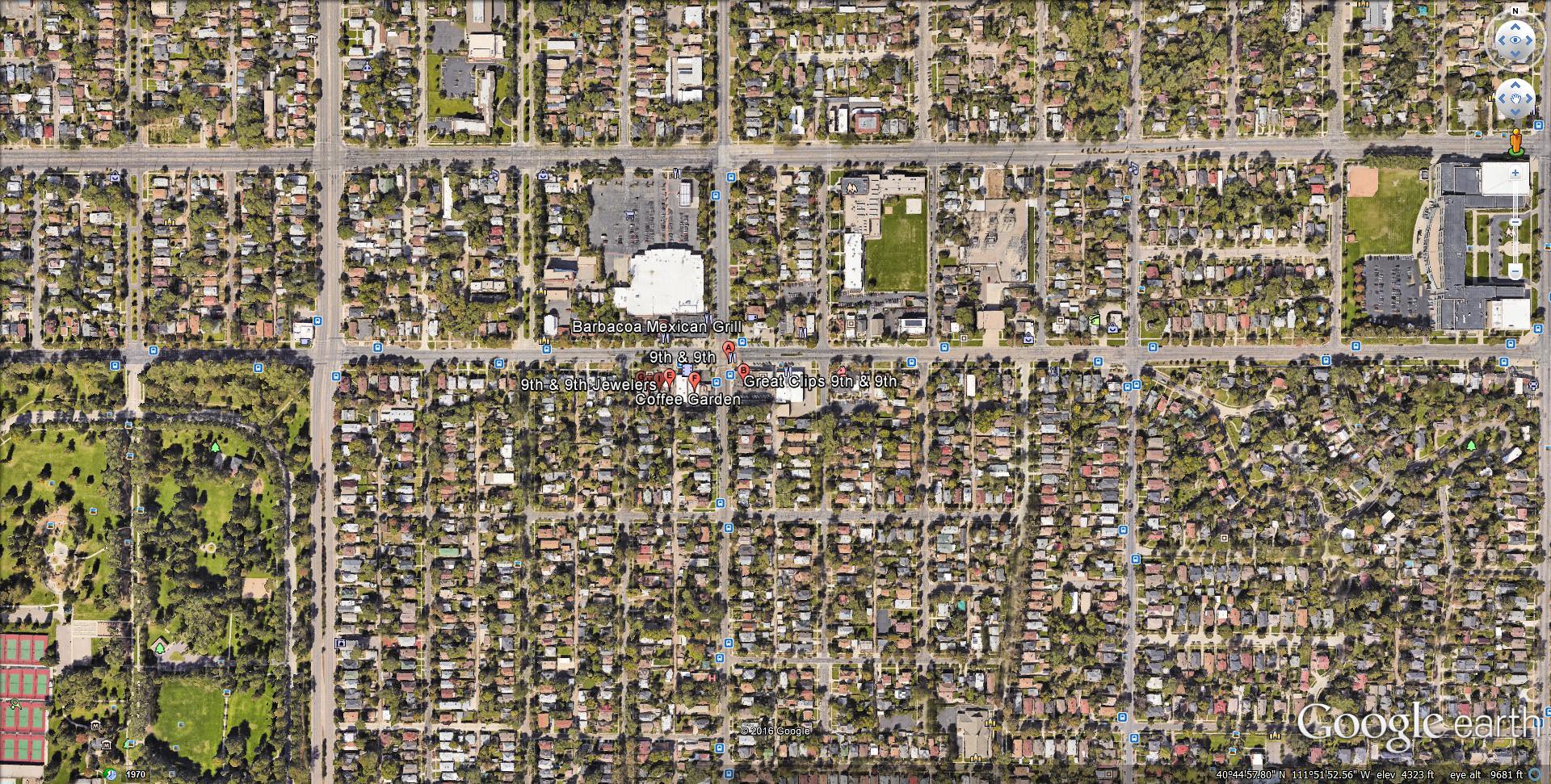A high-resolution Google Earth aerial view captures a sprawling residential area, prominently featuring a white "Google Earth" watermark at the bottom. The panorama exhibits a myriad of houses and buildings, with their roofs forming a mosaic of colors, including gray, brown, tan, terracotta, and black. Verdant patches of green grass punctuate the landscape, some forming part of the yards, while others are isolated expanses showing signs of patchiness and brown spots. Distributed throughout the area, thick, leafy trees provide lush, green canopies.

The image displays a variation of building colors, notably white, but the view is slightly pixelated, making finer details less discernible. Faint white text scattered over the image indicates street names, albeit blurry and hard to read. Notable red and blue pin markings dot the map, marking specific locations. Street layouts are visible on the pavement, adding an organized grid to the scene. At the top of the image, a toolbar features circular control icons with gray and blue arrows for zooming in and out, enhancing navigational ease.